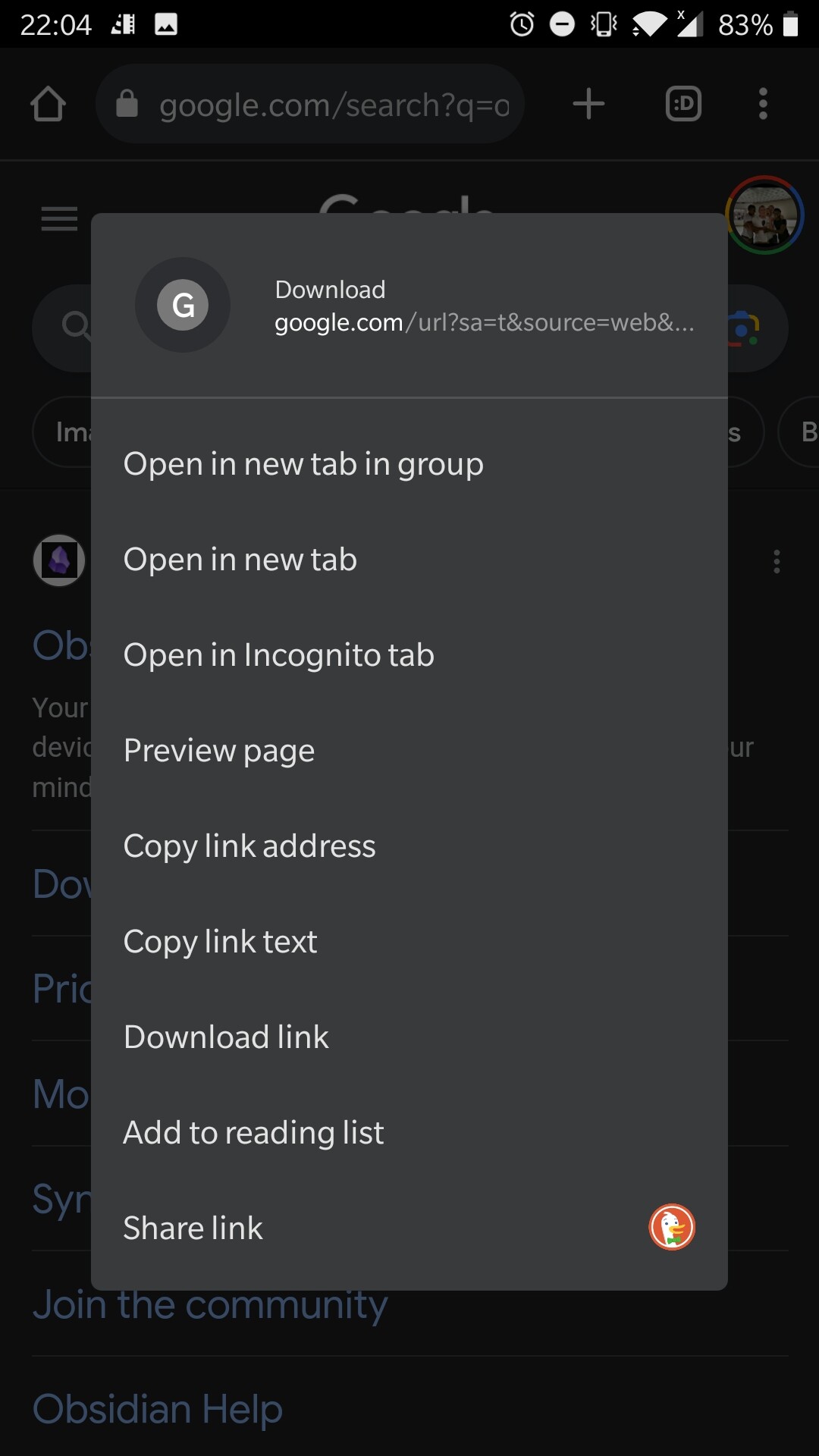This image is a screenshot of a Google search results page displayed in dark mode, characterized by a dark background and white text. Dominating the center of the screen is a large, dark gray pop-up window, partially obscuring the search results. In the top left corner of the pop-up, there is a round, gray icon with a white "G" in the middle, signifying Google. To the right of this icon, the word "Download" appears prominently, followed by the URL "google.com/url" beneath it.

The pop-up window contains a total of nine actionable buttons arranged in a list, each serving a specific function. These options include: 
1. Open in new tab in group
2. Open in new tab
3. Open in incognito tab
4. Preview page
5. Copy link address
6. Copy link text
7. Download link
8. Add to reading list
9. Share link

At the bottom right corner of the pop-up, the DuckDuckGo logo is visible, featuring a white duck head inside a circle, set against a dark background. The overall visual theme is consistent with dark mode, offering a subdued and less eye-straining user interface.